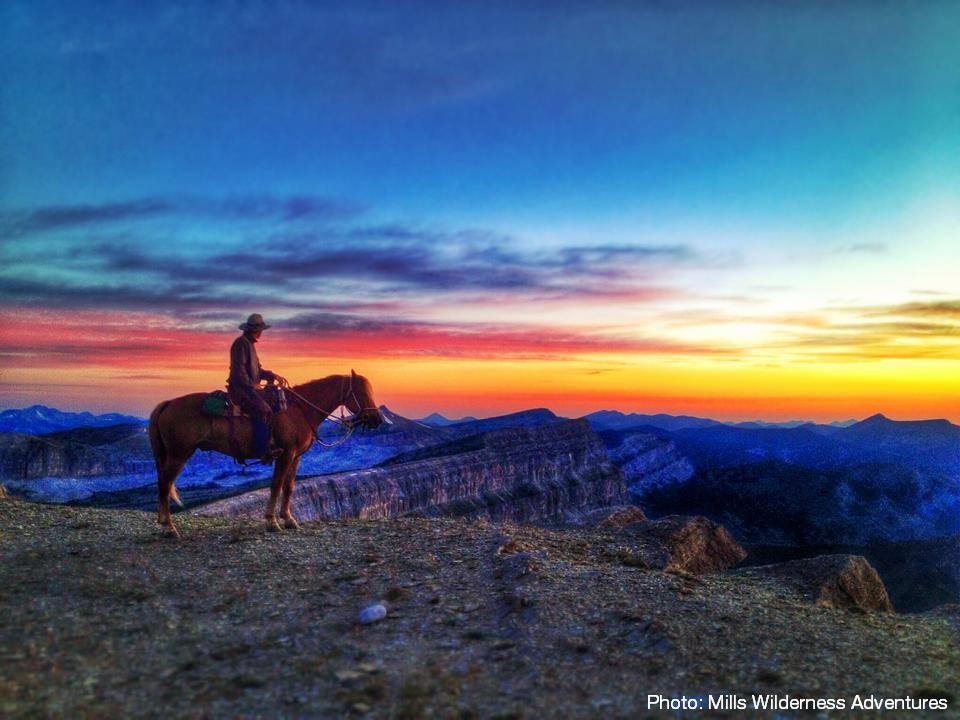This photograph, labeled "Photo: Mills Wilderness Adventures" in white letters at the lower right-hand corner, captures a breathtaking scene at the Grand Canyon. In the foreground, a man wearing a cowboy-style hat sits astride a brown horse equipped with reins and a bridle. They are positioned on a grassy, brown-streaked cliff top, gazing down into the expansive, steep canyon adorned with deep gorges. A stone is visible on the ground nearby. The distant horizon showcases a stunning sunset, with brilliant bands of orange and yellow near the horizon, transitioning into a blue sky dotted with clouds. The far-off mountains and rock formations display a bluish tinge, adding to the image's depth and majesty.